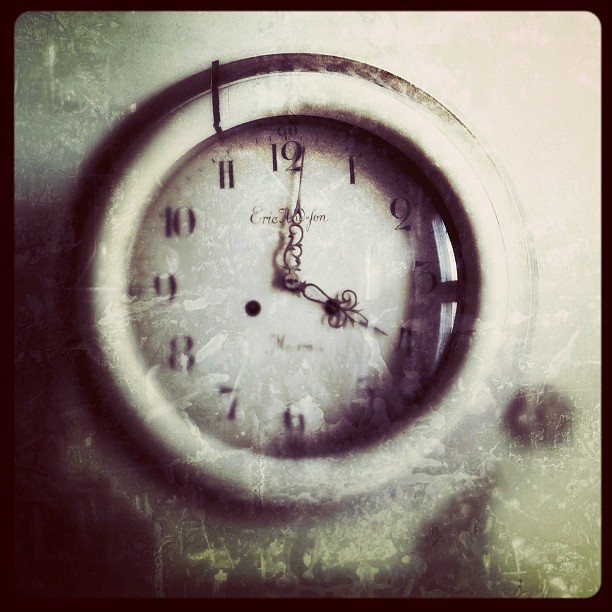The image depicts a rectangular photograph with its length oriented vertically. A black border frames the entire picture. The focus of the image is a wall-mounted clock with a white face and ornate, likely metallic, black hands. The clock’s numbers are also black but appear mostly out of focus except for the numbers 12, 1, and 2, which are prominently sharp. The clock displays the time as 4:01. Just below the number 12, there is partially obscured text, which reads "Eric" followed by an indistinguishable word hidden behind the long hand. The clock is encircled by a large, white border, and the background is a subtle gray hue, providing a gentle contrast to the striking black and white timepiece.